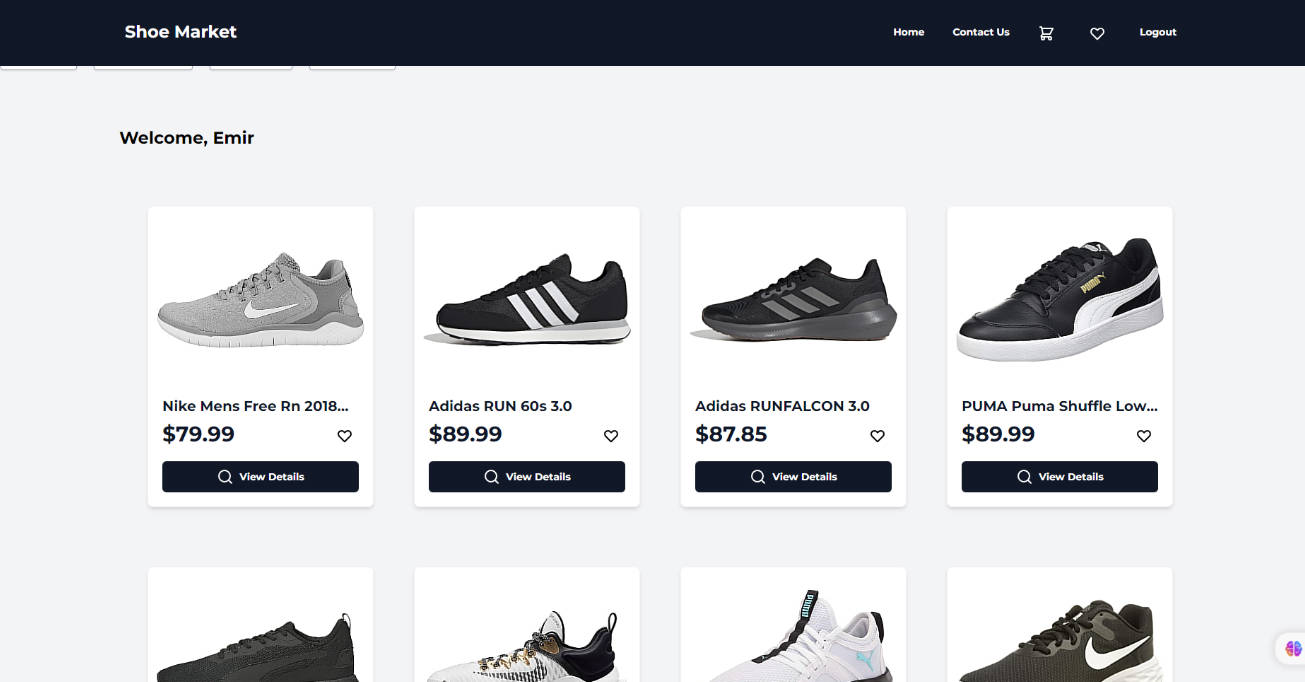The image showcases the homepage of a website named "Shoe Market". At the top of the page, there are several navigation tabs labeled: Home, Contact Us, a Shopping Cart icon, a Heart icon, and Log Out. Below the navigation bar, there is a large banner that says "Welcome". The visible shoe collection is displayed in a grid format, with multiple rows. 

The top row of shoes includes the following models, from left to right:
1. Nike Men's Free RN 2018
2. Adidas Run 60 at 3.0
3. Adidas Run Falcon 3.0
4. Puma Shuffle Low

The background of the website is predominantly white, and the shoes that are visible come in various shades of white, gray, and black. There are additional shoes in the lower rows which are partially visible or obscured.